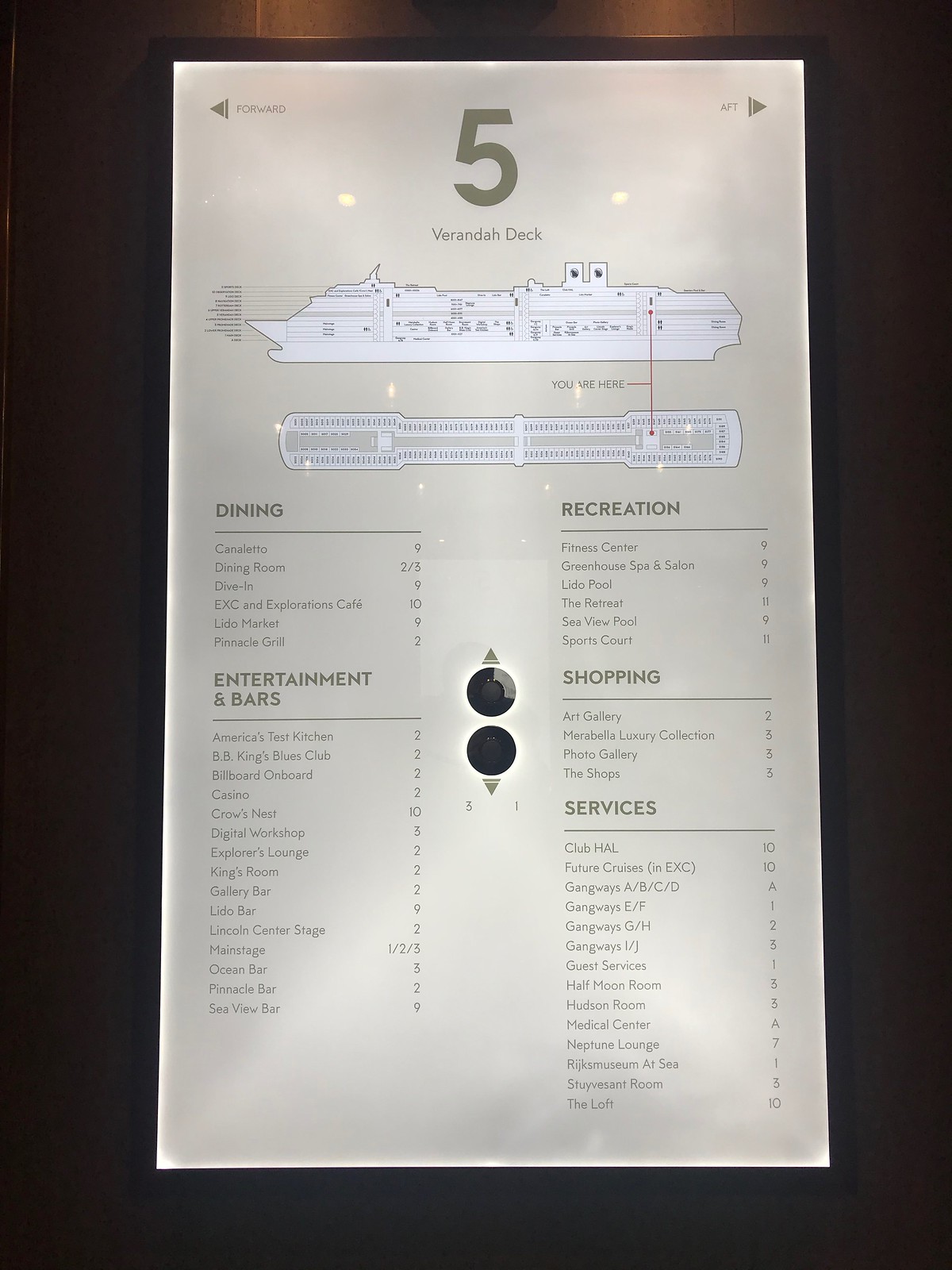This image depicts a detailed map of a cruise ship's deck, likely displayed on an interactive screen. At the top, it identifies the "Veranda Deck 5" and indicates "You are here" to help orient viewers. The map showcases a top-down view of the deck along with labels for various amenities and their corresponding locations on the ship. Notable facilities under the "Dining" section include Canaletto (Deck 9), Dive-In, EXC and Explorations Cafe, Lido Market, and Pinnacle Grill. The "Entertainment and Bars" section highlights BB King's Blues Club, Billboard Onboard, Casino, Crow's Nest, Digital Workshop, and Explorers Lounge. Additional sections cover "Recreation," featuring pools like the Lido Pool and Sea View Pool, a fitness center, and the Greenhouse Spa and Salon (Deck 9). "Shopping" lists venues such as an art gallery, Marabella Luxury Collection, and various shops. "Services" provide information on essential facilities including the guest services desk, medical center, and Neptune Lounge. An interactive touch screen feature is suggested by the presence of scrolling buttons, enabling users to navigate through different parts of the ship's map.